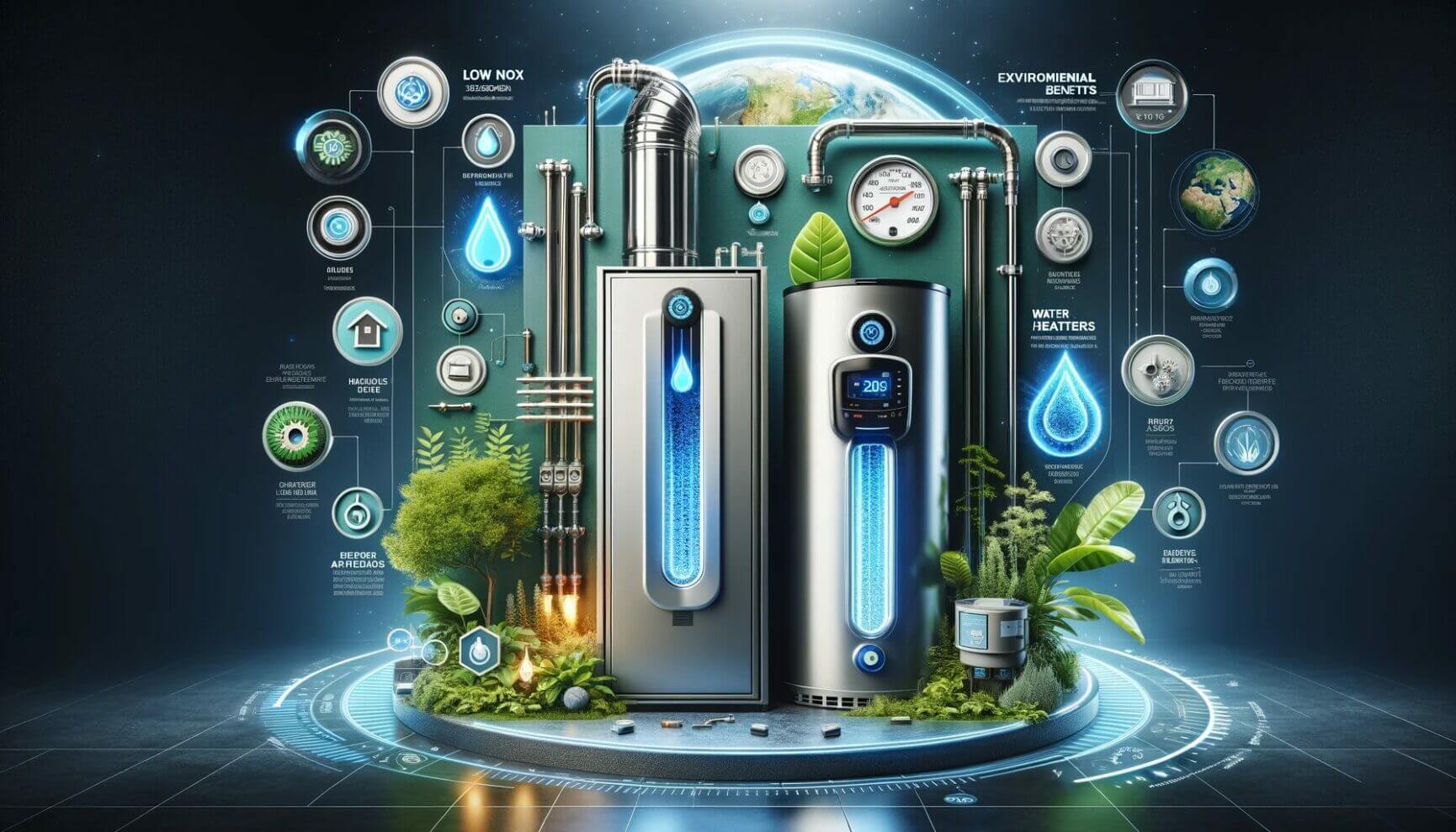The image is a computer-generated, rectangular illustration that appears to be set in a futuristic or virtual environment. It prominently features two main objects in the center, which seem to be water heaters. The object on the right is a tall metallic cylinder with a digital screen displaying the number 209 in blue, accompanied by a black gauge with a white background and a red needle above it. The object on the left is a tall, rectangular unit showcasing a water droplet symbol and a blue line, with a large pipe emerging from its top. Both units have slits indicating water flow and are positioned on a circular metal base surrounded by scattered rocks and plants.

Flanking these central objects are multiple informational bubbles—small circular icons displaying text and images. On the right side, some of these bubbles include text like "Environmental Benefits" and "Water Heaters," while the left side features text such as "Low NOx." However, much of the fine print in these bubbles is too small to discern. The backdrop includes a teal wall with a large green compartment and a pressure dial behind the water heaters, and the overall color scheme includes shades of black, charcoal gray, blue, and green. The ground beneath the objects features a black grid pattern accented with thin white lines. The scene suggests themes related to climate, sustainability, and environmental technology.